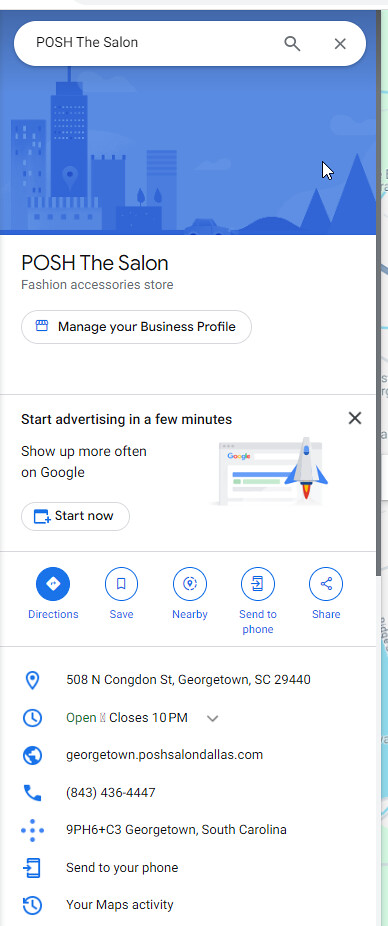A detailed screen capture of a smartphone displaying information about "Posh the Salon" fashion accessories store. At the top is the search bar with "Posh the Salon" entered. Below, a blue box with a stylized cartoon cityscape is visible. The business information is presented underneath. There is an option to manage the business profile followed by a prompt, "Start advertising in a few minutes. Show up more often on Google. Start now." Further down, options for interacting with the business are available, including "Directions," "Save Nearby," "Send to Phone," and "Share." The store's address is listed as 508 North Congdon Street, Georgetown, South Carolina 29440. The screen also provides the store's hours, web address, and phone number.